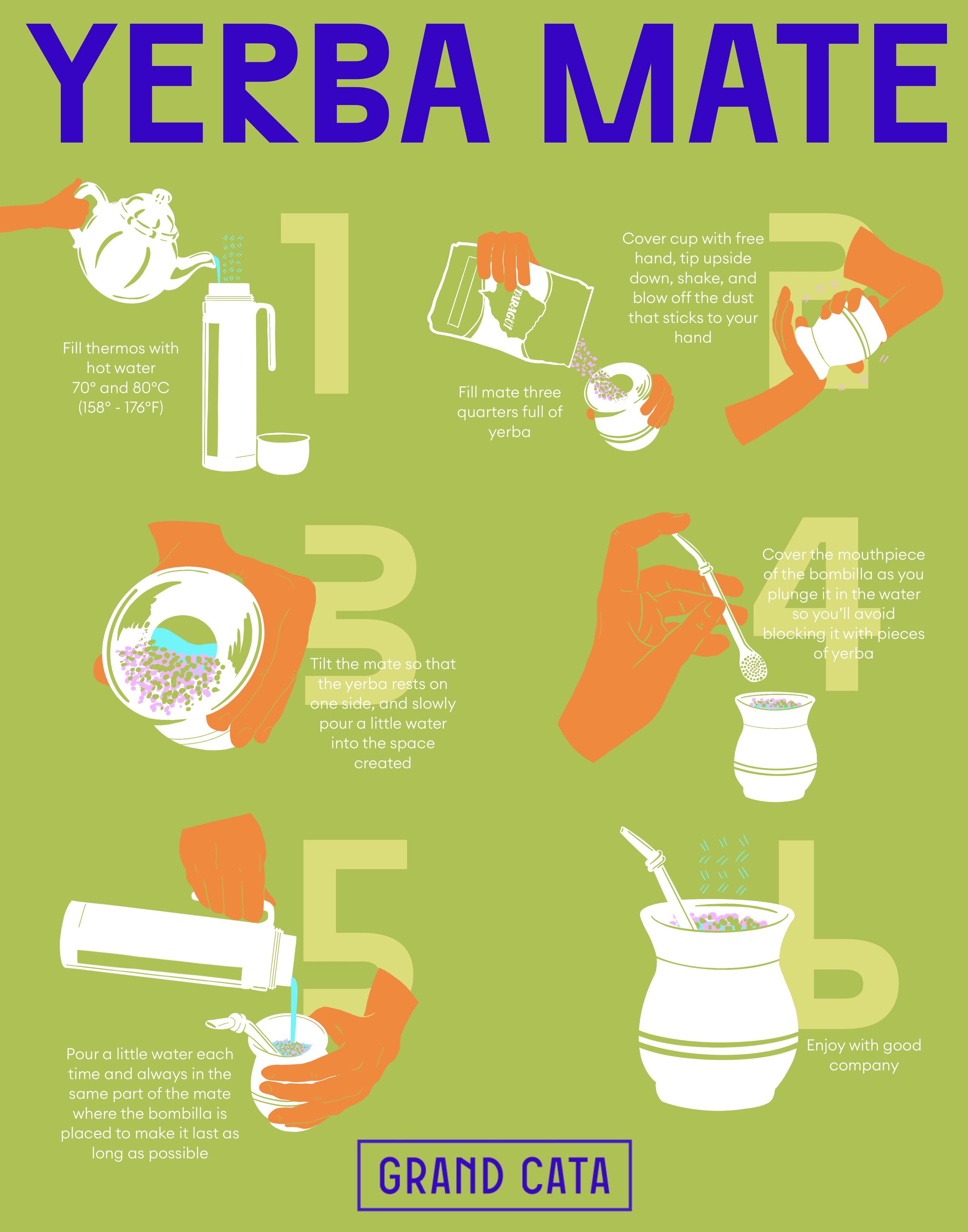The poster features a detailed visual guide on how to prepare Yerba Mate, set against an olive green background. At the top, large blue text spells "YERBA MATE." The steps are illustrated with images and numbered from 1 to 6, alternating between the left and right sides of the poster. 

Step 1, in the upper left, shows a hand pouring hot water from a kettle into a thermos and includes text indicating to fill the thermos with hot water between 70-80°C (158-176°F). 

Step 2, in the upper right, depicts a hand filling a mate cup three-quarters full with Yerba, covering the cup with the other hand, turning it upside down, shaking, and blowing off any dust. 

Step 3, located below Step 1, involves some white text and an illustration of further preparation stages. 

Step 4, below Step 2, shows a hand using a spoon to either add to or take something from a small white jar. 

Step 5, below Step 3, illustrates a hand pouring liquid from a thermos into a cup held by another hand. 

Step 6, below Step 4, displays a white cup with a straw, emanating green lines that may indicate heat or steam. 

At the bottom, a blue-outlined rectangle contains the blue text "Grand Cata." The poster is highly detailed, combining text and images to clearly explain each step of preparing Yerba Mate.